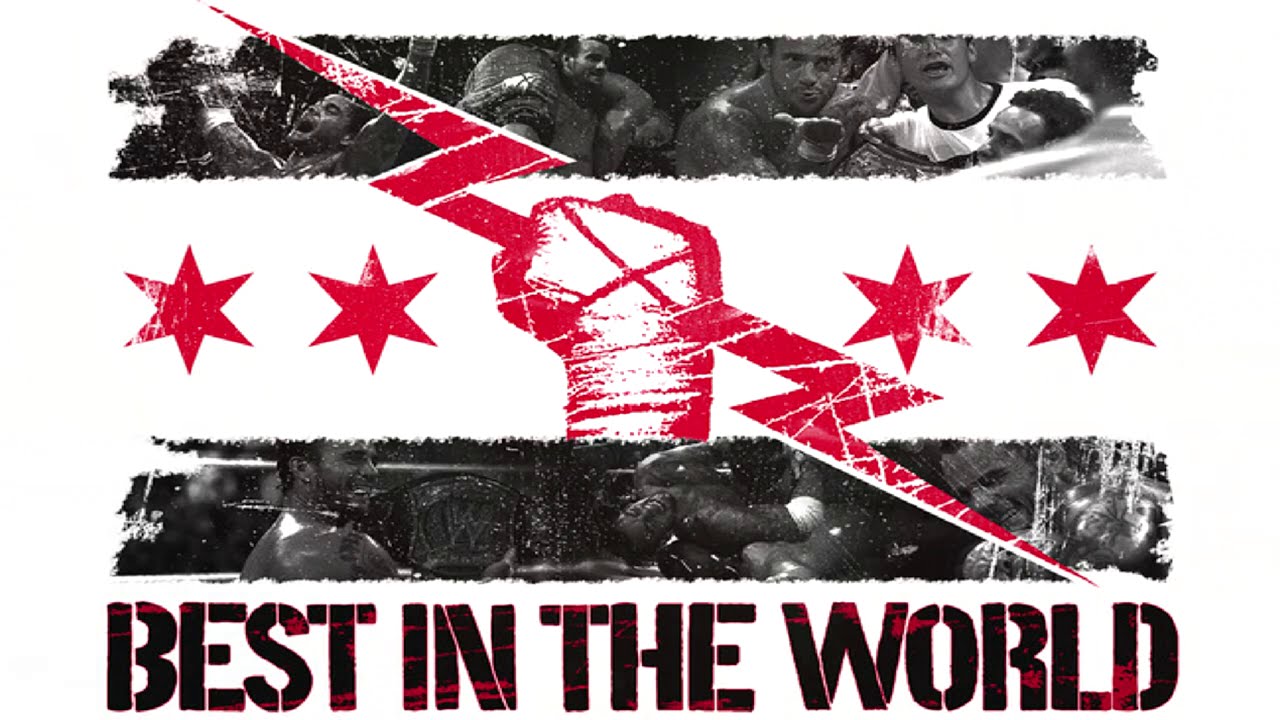The image is a poster featuring CM Punk's logo, prominently displaying his "Best in the World" slogan. The poster is divided into three horizontal sections. The top and bottom sections each have a gray stripe containing black and white images of men wrestling, showcasing CM Punk in various matches and moments from his career. The middle section has a solid white background with a central red fist clutching a lightning bolt, flanked by two red stars on either side. At the very bottom of the poster, the phrase "BEST IN THE WORLD" is written in bold black font highlighted with red accents, emphasizing CM Punk's celebrated status in the wrestling world.